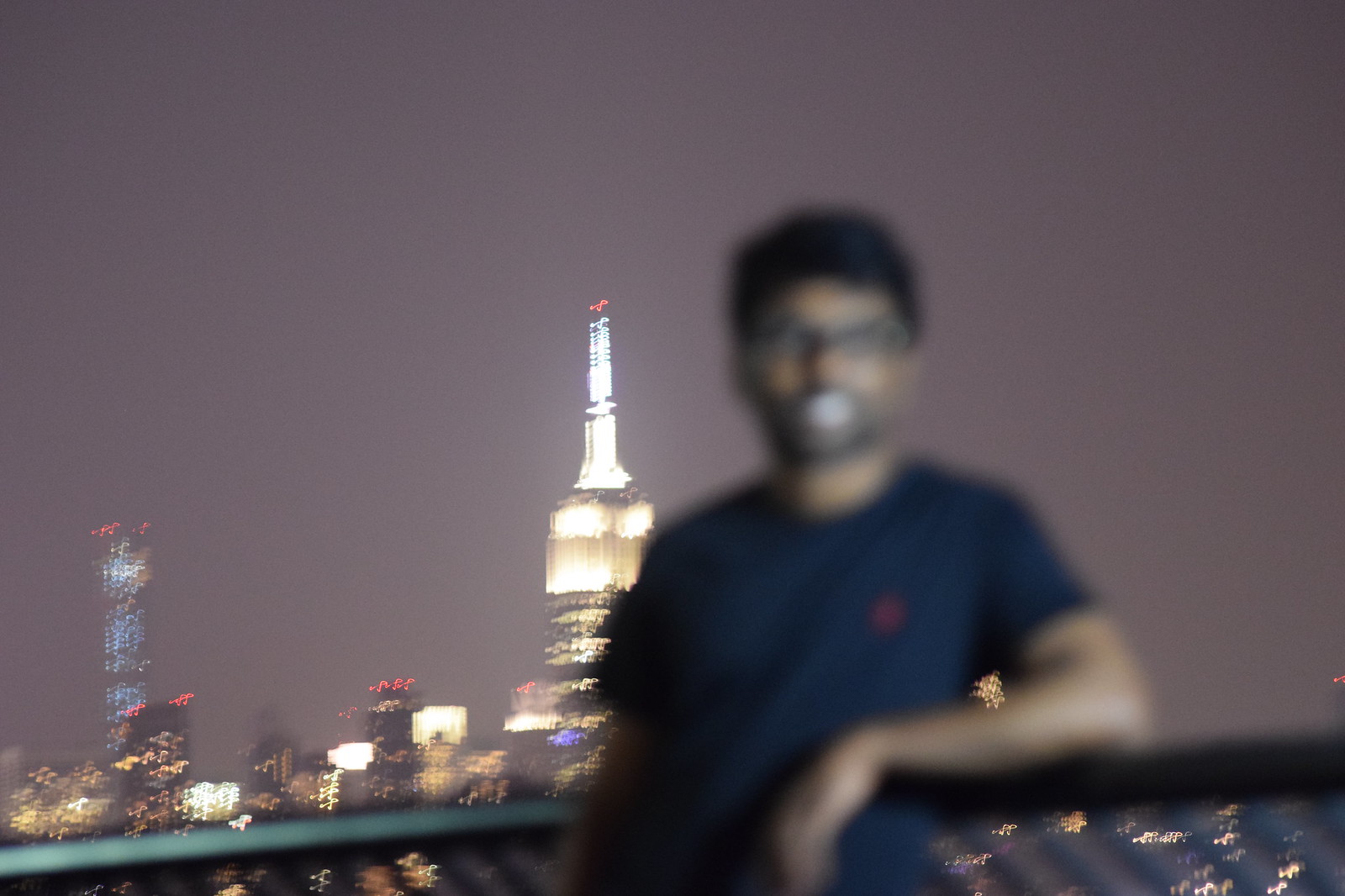In this nighttime image, a man is posed in the foreground with a cityscape behind him. He has black hair, wears glasses, and is dressed in a black shirt. He is leaning casually on a black fence with his left elbow, and he is smiling, showing his teeth. The city skyline behind him is vibrant and illuminated, with a particularly striking tall tower featuring a bright, pointed top adorned with white lights. The base of the tower and surrounding buildings exhibit a mix of yellowish lights, giving them a warm glow. On the left side of the image, another building stands out with its blue lights, while small red lights are dotted around various parts of the scene, adding to the urban nightscape ambiance. Despite the overall darkness, the brightly lit buildings cast a soft glow into the night sky, highlighting the energy of the city.